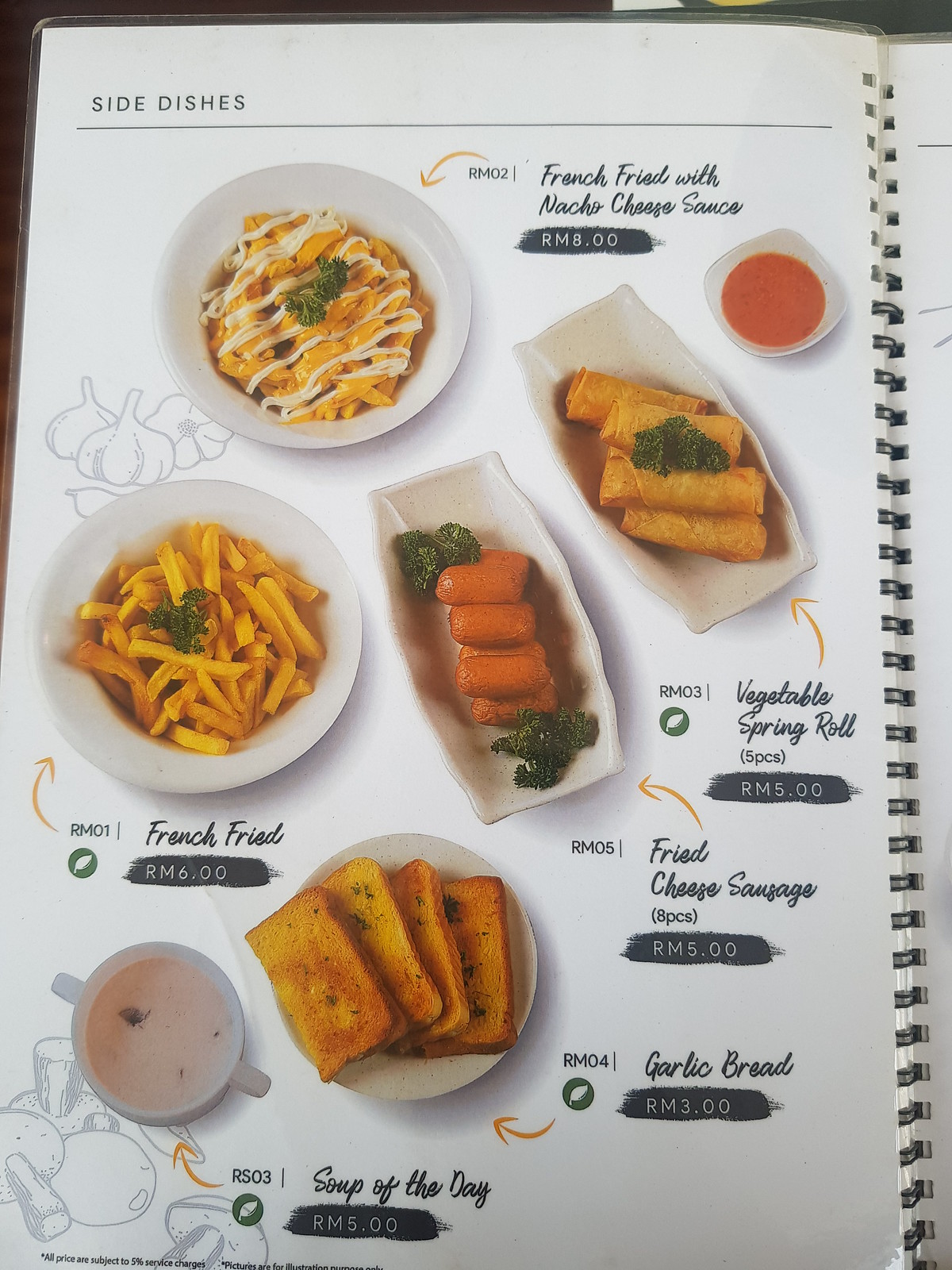The image captures the left side of a two-page menu booklet, showcasing a section titled "Side Dishes." The design is clean and minimalist, featuring a white background with subtle illustrations of fruits and vegetables. Overlaying these illustrations are crisp, real photographs of various menu items, each accompanied by a black box containing the item's name and price.

At the top of the page, the section name "Side Dishes" is prominently displayed. The dishes are organized in a top-to-bottom, left-to-right manner, making them easy to read despite their informal arrangement. Each item is clearly marked with a yellow arrow pointing to its corresponding photograph. The items listed include:

1. **French Fries with Nacho Cheese Sauce** - RM8
2. **Regular French Fries** - RM6
3. **Fried Cheese Sausage** - RM5
4. **Vegetable Spring Roll** - RM5
5. **Garlic Bread** - RM3
6. **Soup of the Day** - RM5

The layout ensures clarity, with ample space around each dish, making it straightforward to identify and select the desired side dish.